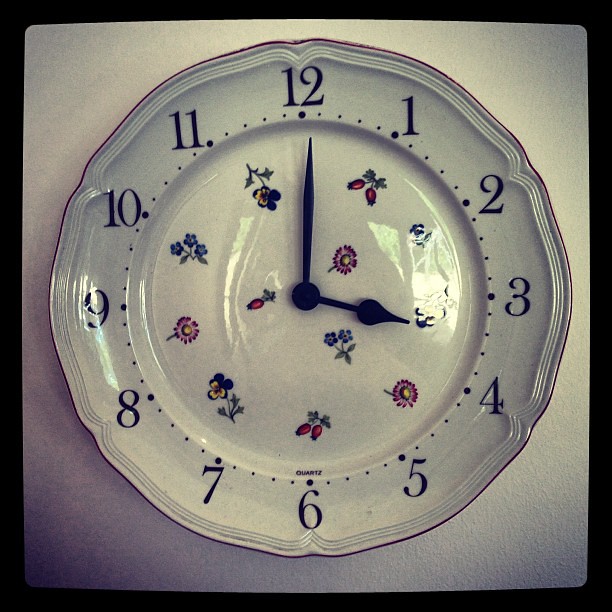This close-up color photograph showcases an exquisitely designed wall clock. The clock's surface resembles a delicate porcelain dinner plate, adorned with ornate silver edging that adds a touch of elegance. Intricate, muted floral patterns featuring soft reds and greens are delicately painted near the center, lending an air of vintage charm. The clock is analog, displaying traditional numbers for each hour from 1 to 12. Its simple black minute and hour hands are positioned to indicate the time as precisely 4 o'clock.